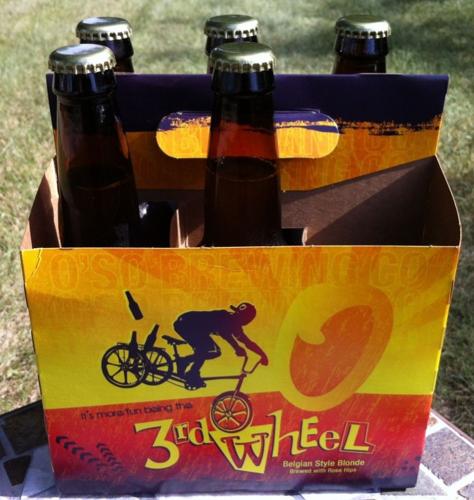This square outdoor photograph, taken on a sunny day, features a close-up view of a six-pack of Belgian-style blonde beer, though only five bottles remain as one is missing. The setting suggests a grassy area with shadows indicating overhead trees filtering sunlight. The packaging is predominantly yellow at the top with a red bottom half. Prominent on the red bottom part in a distinctive yellow and black font is the name "Third Wheel," along with smaller text reading "Belgian style blonde.” The packaging displays an image of a person on a tricycle, wearing a cap, with three brown bottles in the rear basket, one of which is depicted flying out. The box also features a convenient oval handle cutout at the top and is branded with "O'so Brewing Company."